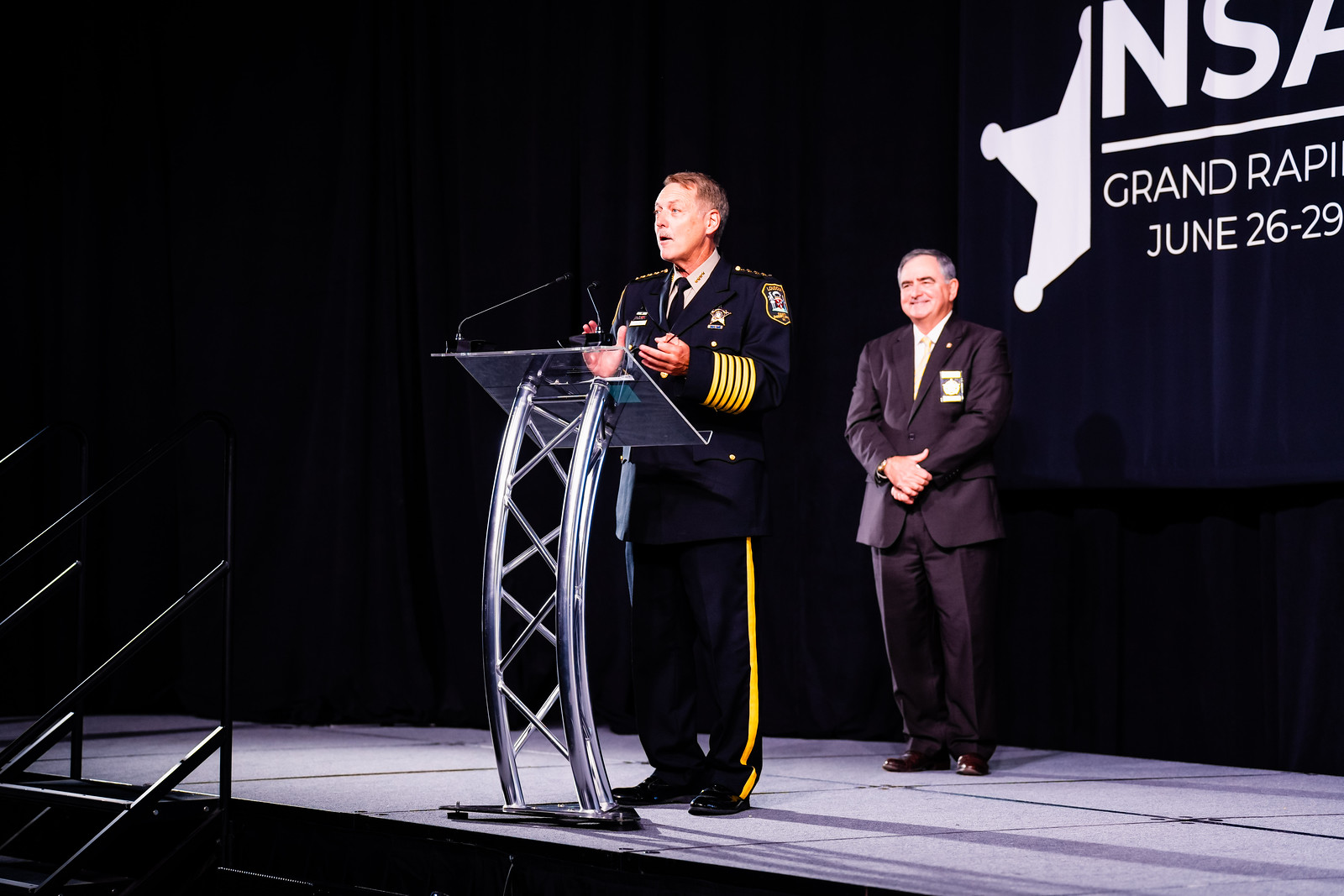The image captures a scene at an event titled "NSA Grand Rapids, June 26-29," visible on a light-colored stage with stairs and a black railing. At the center, a man in military or police attire, identified by his all-navy uniform with yellow stripes or rings on the left arm and down the pants, stands at a clear podium with a chrome, grid-style base. He appears to be in his 50s or 60s with short hair and is in the middle of delivering a speech, with his mouth open and a black microphone in front of him. Behind him stands another man in formal attire, wearing a dark gray or black suit, a yellow tie, and brown shoes, with his arms crossed and smiling. The backdrop features partial text indicating the event's name, location, and date, along with a white badge logo.